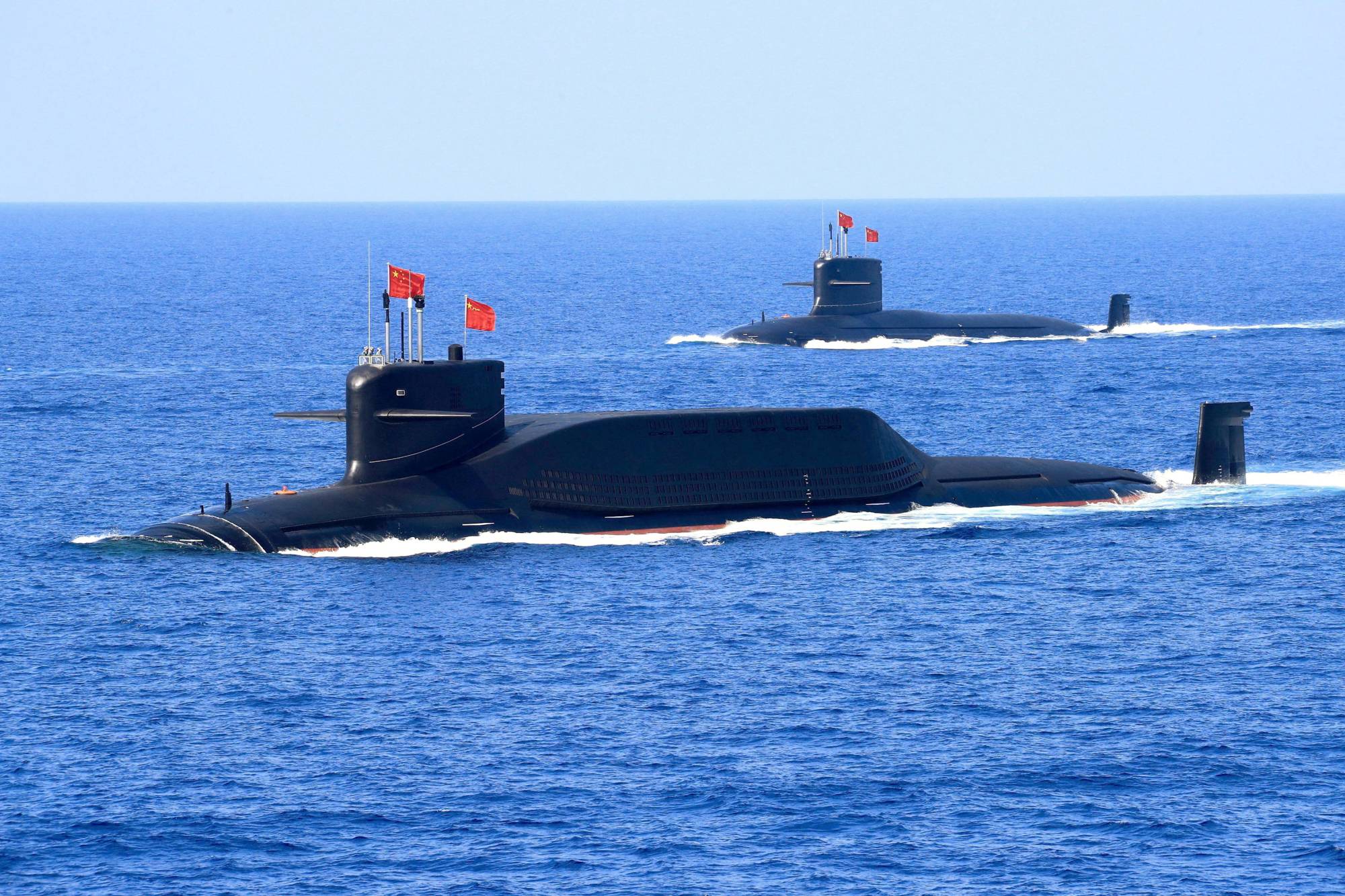In this vividly detailed outdoor image, two submarines can be seen partially submerged in the vibrant blue ocean, their blackish-gray hulls cutting through the ripply water. Each submarine features two small flags with a reddish-orange hue on top, which could be interpreted as either Chinese or possibly Soviet CCCP insignias. The submarines create foamy white trails in the water as they move, leaving behind visible white caps and waves. The scene is illuminated by excellent natural lighting, showcasing an utterly clear, pale blue sky devoid of clouds, and a sharp horizon line separating the ocean from the firmament. The submarines, positioned one in the foreground and the other further back, are set against this serene seaside backdrop, rendering a high-quality and crystal clear photograph.